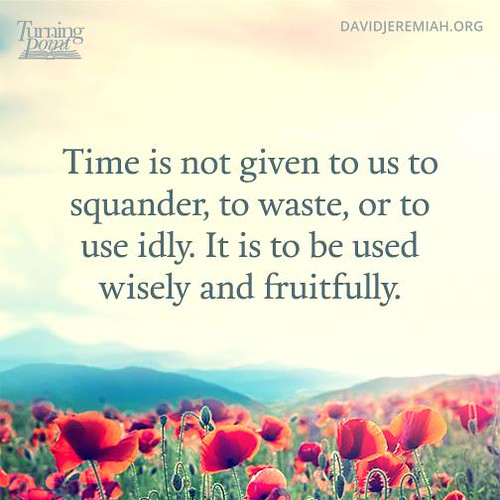This is a detailed and evocative postcard provided by davidjeremiah.org, likely designed for sharing on platforms like Instagram due to its square format. The centerpiece of the image is an inspirational quote set against the backdrop of a picturesque natural scene: "Time is not given to us to squander, to waste, or to use idly. It is to be used wisely and fruitfully." The background depicts a vibrant field of poppies in shades of red and orange with lush green stems. Beyond the flowers, silhouettes and shadows of towering mountains stretch across the horizon, some shrouded in mist. The sky above transitions through a gradient of soft pink, yellow, and blue, enhancing the serene atmosphere of the setting sun. The upper corners of the postcard feature the logo "Turning Point" on the left, resembling an open book, and "davidjeremiah.org" on the right, both subtly reminding viewers of the source of this motivational message. The overall aim is to encourage the viewer to use their time wisely, emphasizing the fleeting and precious nature of every moment.